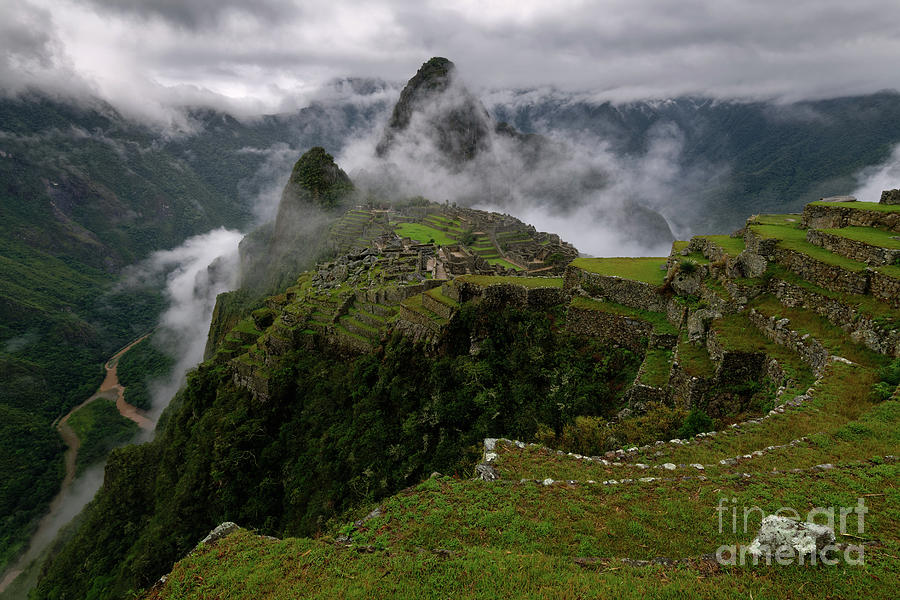This picturesque scene captures the lush, verdant landscape of a mountainside that could very well be Machu Picchu in Peru. The image, branded with Fine Art America in the right corner, displays a complex interplay of natural and historical features. Dominating the foreground is a series of steep, stair-like rocks adorned with greenery. These terraces cascade down the mountainside, leading the eye toward what appears to be an archaeological site, consisting of multiple stone structures and ruins reminiscent of the ancient Incan citadel.

The backdrop is equally mesmerizing, with an expansive range of mountains enveloped by a thick blanket of clouds that seem to descend into the valleys below. These clouds mingle with the high elevation greenery, creating a misty, ethereal atmosphere. To the left, a split off lake or river glistens in the distance, winding through the valley. It's a cloudy yet luminous day, enhancing the vibrant greenery of the trees and vegetation that carpet the mountains and valleys alike. This well-preserved site, with its multiple levels and historical significance, is a visually stunning destination, perfect for sightseeing and absorbing the grandeur of an ancient civilization amidst breathtaking natural beauty.